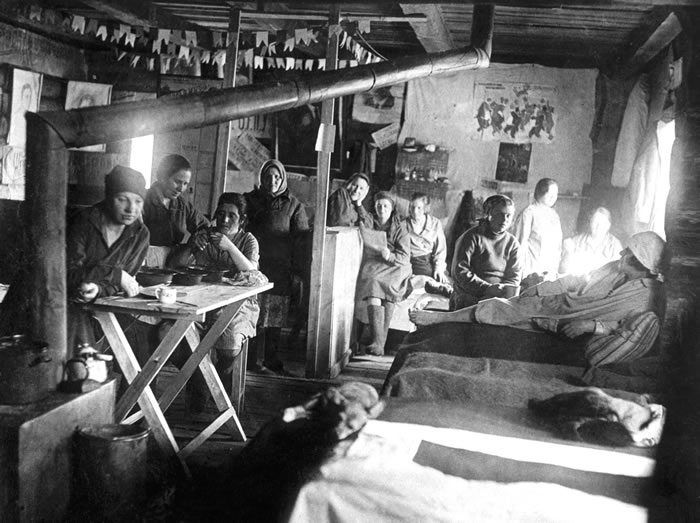The black and white photograph appears to be taken inside a small, dimly lit room from the early 19th century, featuring a somber, communal atmosphere. The cramped interior shows 11 women gathered, possibly indicating a group home or a makeshift shelter for the poor. The room is sparsely furnished, with beds lined along the right wall, their footboards pointing towards the room's center. Additional beds may be positioned along the far wall. One woman is seen lying on a bed, wearing old-fashioned pajamas and a night cap. Near the room’s center, two women sit at a small, rustic wooden table with crossed legs. The women in the room are dressed warmly, in coats, scarves, and hats, suggesting a need for warmth and adding to the downtrodden impression of the scene.

A wood-burning stove, identified by its prominent piping that extends upward before angling across towards the ceiling, occupies a corner, suggesting the need for warmth in this impoverished setting. The walls bear a few posters or paintings, though the room lacks any suggestion of wealth or comfort. Two windows on opposite walls allow for some natural light, but the overall ambiance indicates a lack of affluence. The homemade furniture and overall conditions hint at a humble, struggling existence during a challenging period.